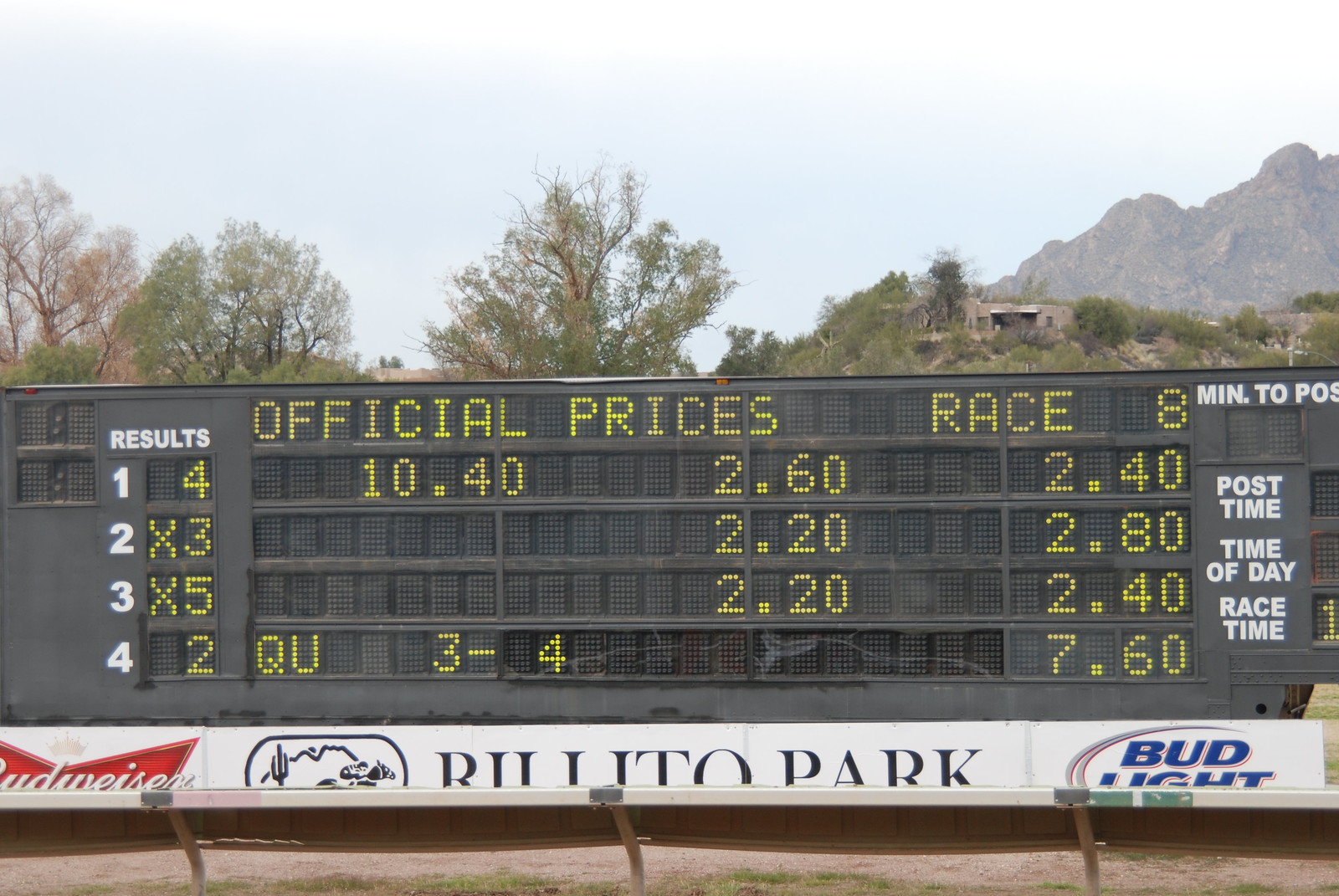This image captures an expansive, horizontally-oriented black digital scoreboard at a racetrack, prominently displaying the "Official Prices Race 8" in bright, yellow digital text. The board's left section lists results in both yellow and white text, including positions one through four, while to the right, it displays crucial racing information like post time, race time, time of day, and minutes to post in white. The digital display also shows various betting amounts and outcomes, such as "$10.40, $2.60, $2.40, $2.20, $2.80, $2.20, $2.40, QU 3-4, $7.60." At the bottom of the scoreboard, a white sign features the Budweiser logo on the left, the Bud Light logo on the right, and center text likely indicating "Bill Ito Park," partially obscured by a barricade that perhaps separates the track. In the background, vibrant green trees are in full bloom under a gray sky, with a rocky mountainous area and a brown house perched atop a cliff adding depth to the scene.